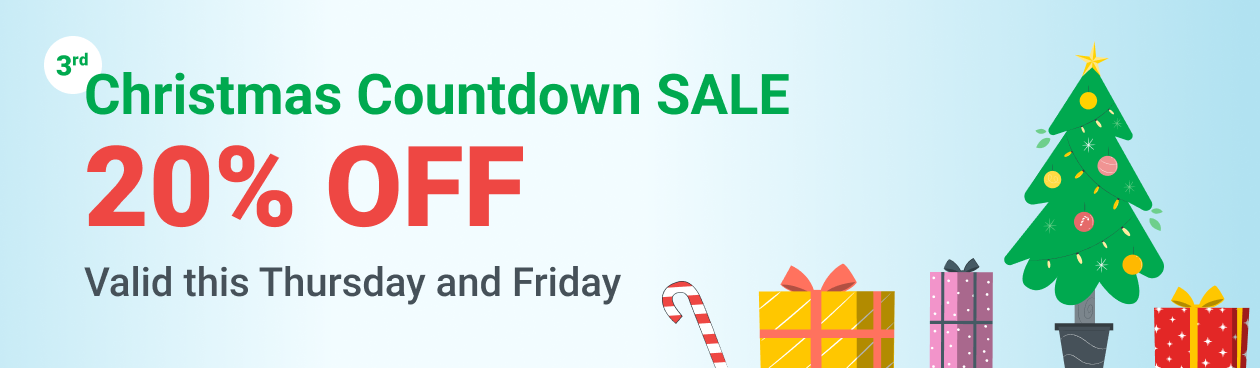The image features a gradient background transitioning from light blue on the left, blending to white in the center, and shifting to a darker blue on the right side. In the upper left corner, a white circle with the number "3" inside and the small letters "RD" above it signifies "3rd". Below this, in bold green text, the words "Christmas Countdown Sale" are prominently displayed, with "SALE" in uppercase. Beneath this, "20% OFF" is written in bold red print. Further down, in black print, it states "Valid this Thursday and Friday."

On the right side of the image, there is a series of festive elements. Starting from the left, there is a red and white striped candy cane, approximately three inches tall. Next to it is a yellow-wrapped present with a red bow and ribbon. Further to the right, there is another present, about four inches tall, wrapped in pink paper with white dots and adorned with a navy blue bow. Adjacent to this is a small Christmas tree, approximately five to six inches tall, displayed in a black pot. The tree is green with pink and yellow ornaments and topped with a yellow star. Finally, on the far right, there is another present wrapped in red paper with a yellow bow.